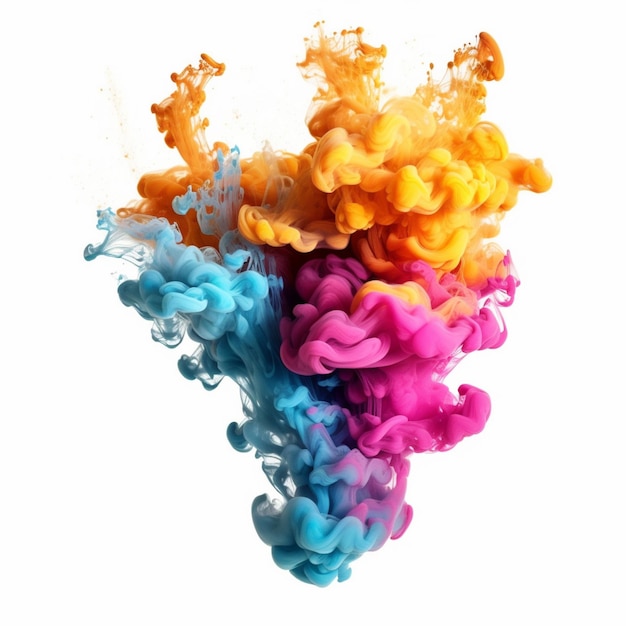The image showcases a vibrant, psychedelic blend of colors in a form that evokes the appearance of swirling gases or smoky plumes. Against a plain white background, several distinct hues merge and interact. To the far left, deep blue flows upward, with some streaks extending towards the center. Moving rightward, the colors transition to a vivid pink that prominently occupies the front and center of the image. The pink area appears to fuse with the blue towards the bottom, creating a dynamic mix before settling into their respective colors again.

Behind the blue and pink, an orange and yellow combination adds warmth, spreading across the upper segments of the image. Notably, above the pink, orange subtly blends in, enhancing the visual complexity. The topmost areas of the composition feature these colors in splash-like patterns, creating an energetic, almost explosive appearance. The overall shape of the colorful formation suggests an upwards expansion, with a visual flow from the smaller base towards broader, more dispersed upper regions, hinting at an arrow-like shape pointing downwards. The interplay of waves and splashes in contrasting hues makes for an engaging and mysterious visual experience.